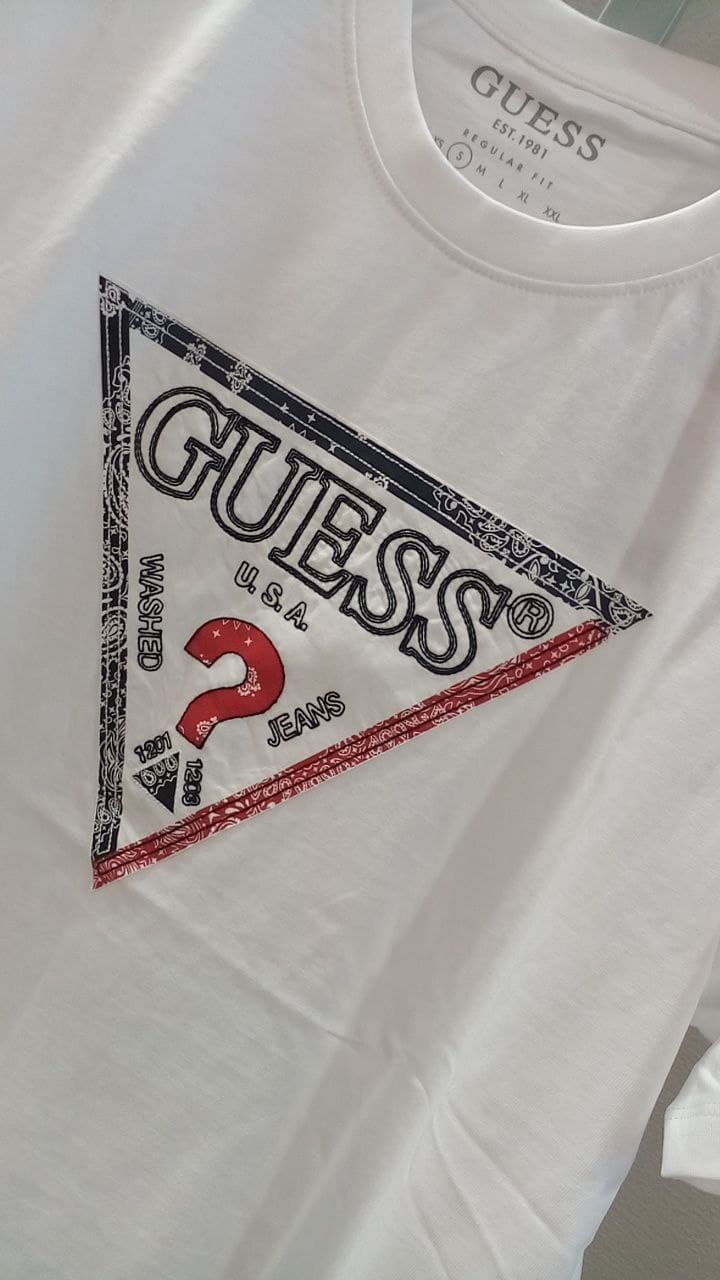This image features a white, short-sleeve Guess Jeans t-shirt. On the front chest area, there is a prominent upside-down triangle design. The border of this triangle features a paisley print in blue and red, reminiscent of bandanas, while the interior of the triangle's border remains white. At the top of the triangle, the word "GUESS" is displayed, followed by "USA" and "WASHED JEANS". Below this text is a red question mark, containing a paisley motif, and the numbers "1201" and "1203". On the back inside collar, the t-shirt reads "Guess Established 1981 Regular Fit Small". The sides of the triangle in the design are black, black, and red, giving it a distinctive appearance. Overall, this designer shirt by Guess Jeans combines classic elements with intricate details.